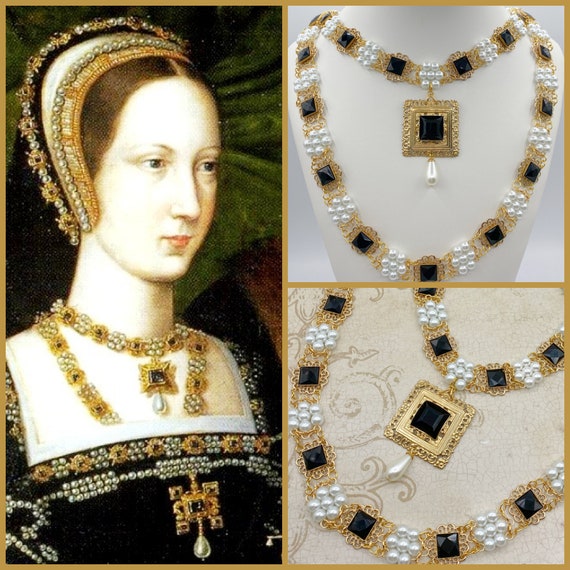This image is divided into three distinct sections. On the left, there's an old portrait of a regal woman, possibly royalty, set against a dark green background. Her pale face is framed by slicked-back brown hair, adorned with an elaborate headpiece made of gold, white, and black materials, intricately decorated with pearls. She wears a large, ornate necklace with a floral design made of pearls, gold, and gems, featuring a central square pendant with a pearl hanging at the center. Her black dress is also embellished with pearls and gold accents. On the right, the image is divided into two square panels displaying close-ups of her lavish necklace. The upper panel highlights the intricate details of the necklace, which is crafted from pearls, gold, and dark gemstones. The lower panel continues to showcase the same necklace, emphasizing the large, square emerald pendant at the center, surrounded by gold and pearls.